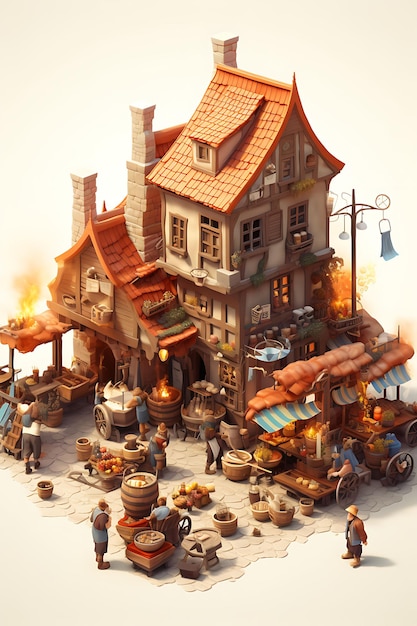This detailed AI-generated image depicts an isometric view of a medieval market square. At the center stands a multi-story building with distinct pagoda-like architecture, reminiscent of Austrian or German styles, featuring steep curved roofs designed for a winter climate. The house, complete with three levels and chimneys on the left, anchors the scene.

In front of this building, a bustling market unfolds. To the right of the house, there is a streetlight beside a truck loaded with various items, including some pots and whiskey barrels positioned to the lower left. A figure stands beside the truck, contributing to the lively atmosphere. Directly below the house sits a cart stand with an awning, displaying candles, baskets, and items arranged on a table. Bushes and other small decorations surround this area.

The left side of the image features an open town square, populated by scattered figures, carts, and a variety of market stalls. One notable cart appears to be serving food. The market is vibrant with activity, including flames rising from barrels, and fruit and vegetables arranged in wooden crates. The entire scene captures the essence of a historic market square, brought to life through vivid colors of orange, gray, brown, light blue, and yellow, all emphasizing the digital rendering's intricate details in this fantasy creation.